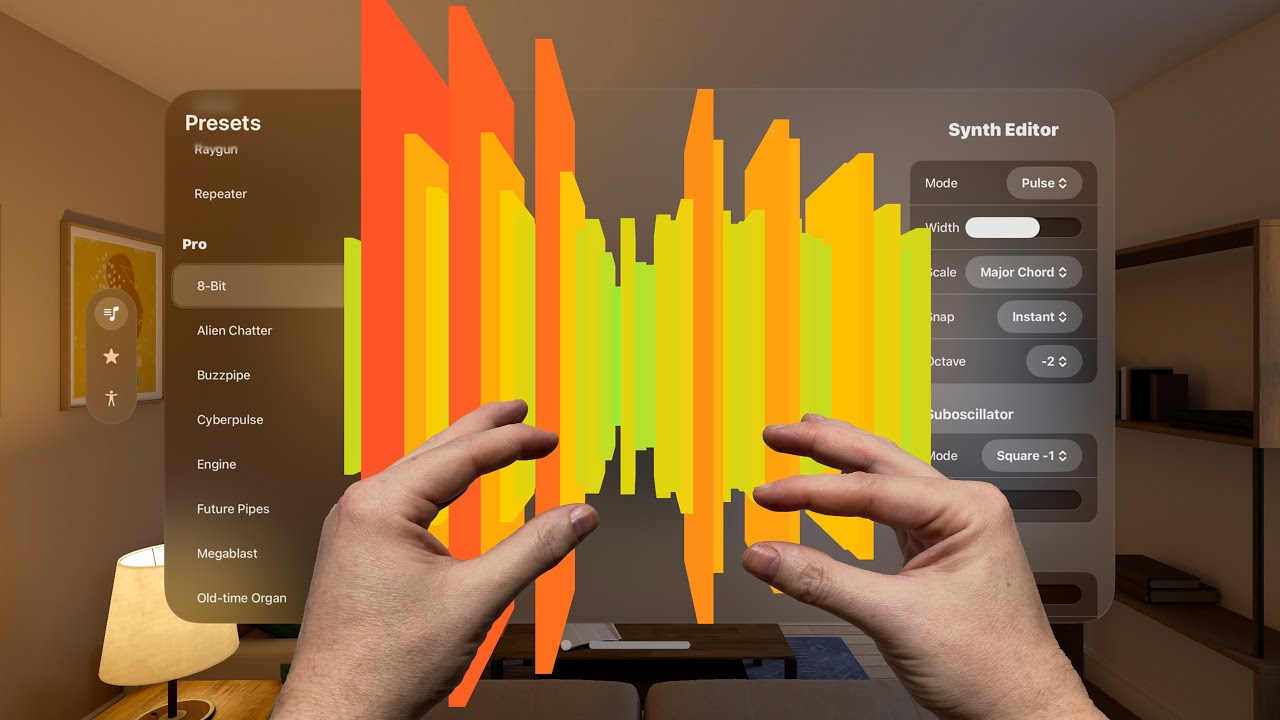The illustration depicts a VR or metaverse interface showcasing an interactive audio recording software. The central focus is a brownish-gray board featuring orange and yellow wave patterns, with a photograph of two human hands interacting with it. On the left side of the board, a column labeled "Presets" displays various settings such as Pro, 8-bit, Alien Chatter, Bus Pipe, Cyber Pulse, Engine, Future Pipes, Mega Blast, and Old Time Organ. The right side is headed "Synth Editor" and includes detailed parameters like Load Pulse, Width, Scale (Major Chord), Snap (Instant), Octave (Negative 2), Subsilitor, Mode (Square, Negative 1). The board and hands are set against the interior of a room with grayish-brown walls. The left wall features a painting and a counter or table with a lamp that has a white shade, while the right wall has built-in shelves. The realistic 3D graphic look suggests a VR environment where users can manipulate the software with hand gestures, highlighting the immersive and futuristic nature of the application.